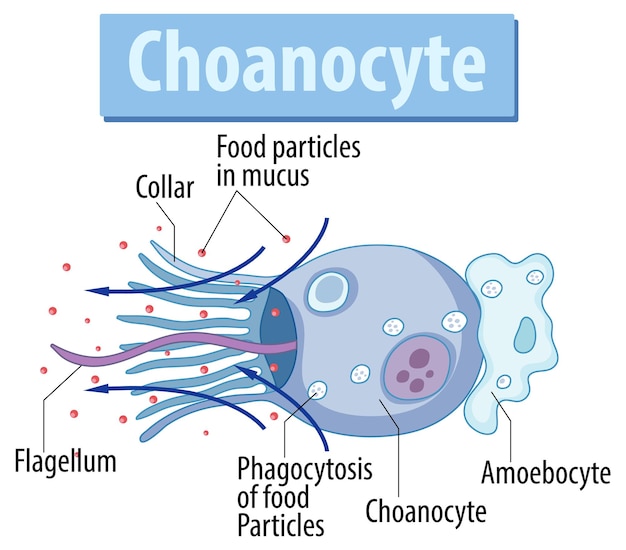This is a detailed illustration from a biology textbook depicting a choanocyte. At the top of the image, a light blue rectangular banner with a darker blue drop shadow prominently displays the word "CHOANOCYTE" in lighter blue font. Beneath the banner lies the main illustration, which features a circular, lighter bluish-gray body resembling a jellyfish or octopus, viewed from the side. This body has several teal tentacles extending outward, with one long, squiggly purple tentacle, labeled "flagellum," emerging from the middle towards the left.

The tentacles, labeled "collar," are surrounded by smaller red dots identified as "food particles and mucus," essential for the cell's feeding mechanism. The main body of the choanocyte is also dotted with smaller white particles. Additionally, a detailed label describes the "phagocytosis of food particles," noting the cell's function in engulfing food. 

On the right-hand side of the main body, an irregularly shaped blob labeled "amoebocyte" is visible, showing another type of cell associated with this structure. This entire scene is meticulously arranged to clearly represent the biological components and functions of a choanocyte, making it an informative diagram for educational purposes.